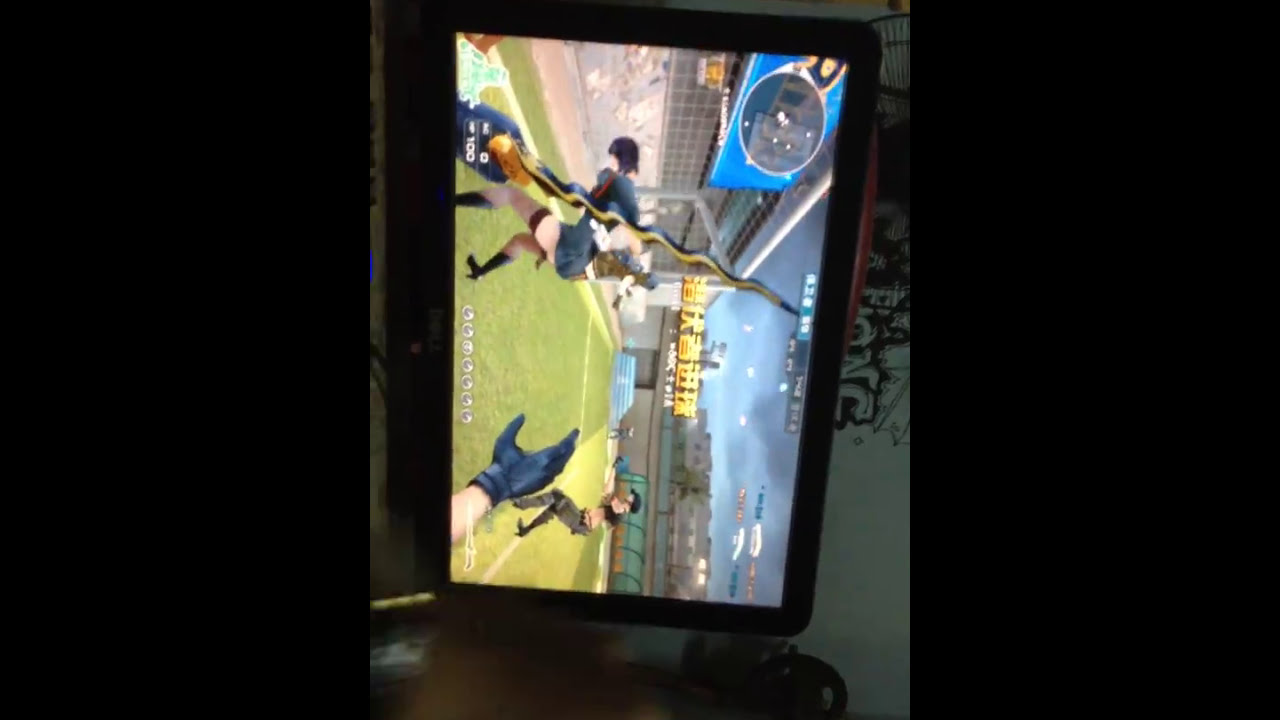The image features a sideways view of a tablet displaying a video game, composed within a frame where black borders occupy the outer two-thirds, leaving the central third to the screen. The game interface is rotated 90 degrees counterclockwise and is cluttered with text in an Asian language, possibly Japanese or Chinese. The graphical scene includes cartoon-like characters seemingly engaged on a soccer or baseball field set inside a stadium. In the foreground, a central character, a woman dressed in a short skirt, hosiery, and high heels, holds a strange squiggly object, resembling a lightning bolt, with dark skies overhead. To her left is another woman bent over, possibly maneuvering a blue bag or backpack, while on the lower right is a hand clad in a black glove pointing forward. The distant background depicts another figure standing amidst surrounding great buildings and stadium structures, completing the scene with an atmosphere of an outdoor sports event under moody skies.